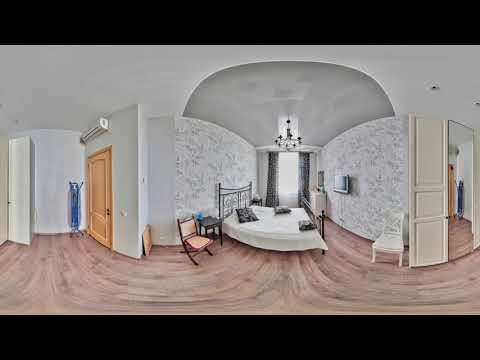The image showcases a neatly arranged bedroom with dominantly white decor, accentuated by intricate details. Central to the room is a steel-framed bed adorned with a white bedspread and three pillows. The surrounding walls are white with soft gray floral or leaf patterns, creating a serene and cohesive backdrop. Above, a chandelier hangs elegantly from the fully white ceiling. 

To the left of the bed is a notable foldable peach or red chair beside a side table. On the opposite side, a white chair stands next to another side table, further complementing the room's minimalist elegance. The floor is a pinkish-brown shade, adding a subtle warmth to the space. 

Noteworthy features include a television mounted on the wall opposite the bed, situated next to a window draped with black curtains. The left side of the room presents a closed brown wooden door, seemingly leading to another hallway or room, evidenced by an ironing board leaning against the wall. On the right, there's an open doorway providing a glimpse into an adjacent space or possibly reflecting a mirror.

This detailed ambiance, captured in a 360-degree view, gives the room a spacious and inviting appearance, reminiscent of a pristine hotel suite.